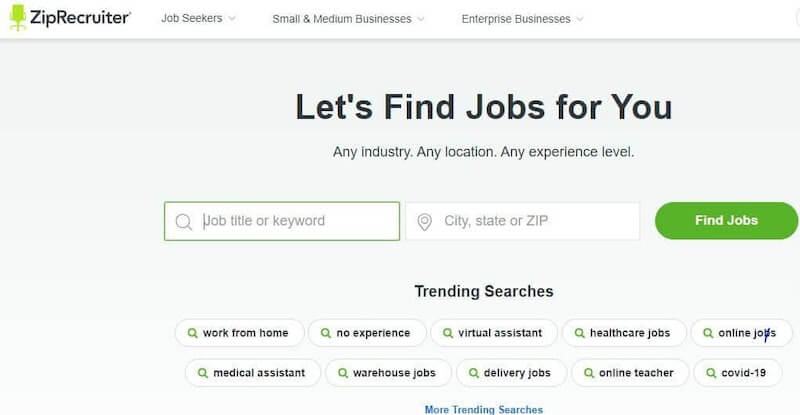Screenshot of ZipRecruiter Homepage:

At the top of the screenshot, three primary navigation tabs are visible: "Job Seekers," "Small & Medium Businesses," and "Enterprise Businesses." Each tab features dropdown menus offering additional options. The main section of the page has a light green background with a prominent black headline that reads, "Let's find jobs for you. Any industry, any location, any experience level."

Below the headline, there are two white search boxes. The left box, which has grayed-out placeholder text saying "Job Title or Keyword," is accompanied by a magnifying glass icon. The right box, displaying "City, State, or Zip" as a placeholder, is marked with a map drop pin icon. A green "Find Jobs" button is situated beneath these search boxes.

Underneath the search section, in slightly smaller text, is the label "Trending Searches." This is followed by various circular thought bubbles containing popular job queries such as "Work from home," "No experience," "Virtual assistant," "Healthcare jobs," "Online jobs," "Medical assistant," "Warehouse jobs," "Delivery jobs," "Online teacher," and "COVID-19." Additionally, a "More Trending Searches" link is shown in blue at the bottom of this section.